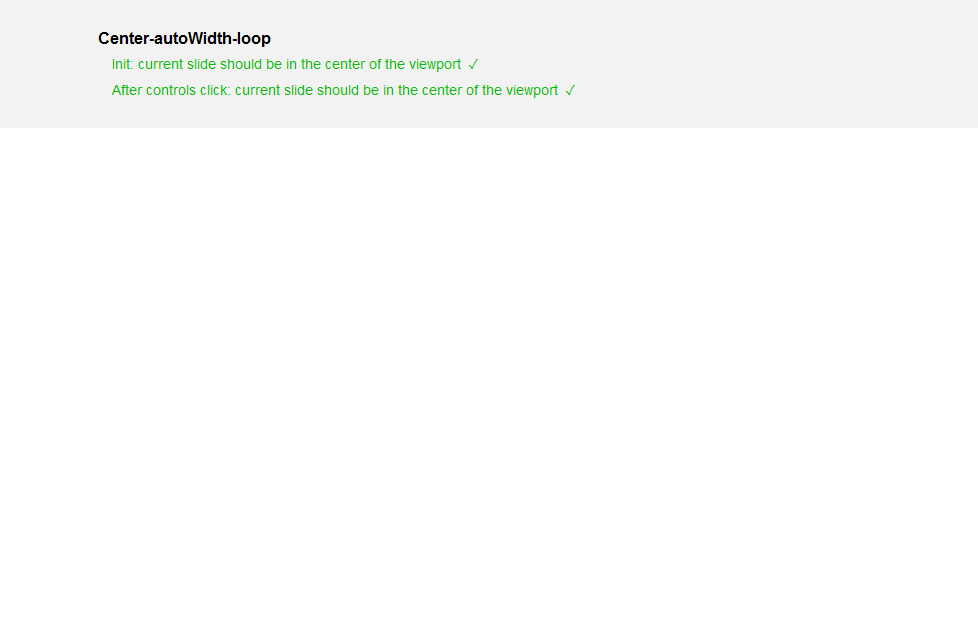Image Caption: 

The image features a minimalistic gray background. Positioned on the left side, the black text reads "Center-Auto Width" with capitalized 'W' and is followed by "-Loop." Directly below this, in green text, it states "init." (short for initialization), indicating that the current slide should be centered within the viewpoint, accompanied by a small green check mark. On the next line, also in green text, it reads: "after controls click, current slide should be in the center of the viewpoint," again marked with a green check mark. The overall design is simple and straightforward, focusing on conveying the alignment status of a slideshow element.